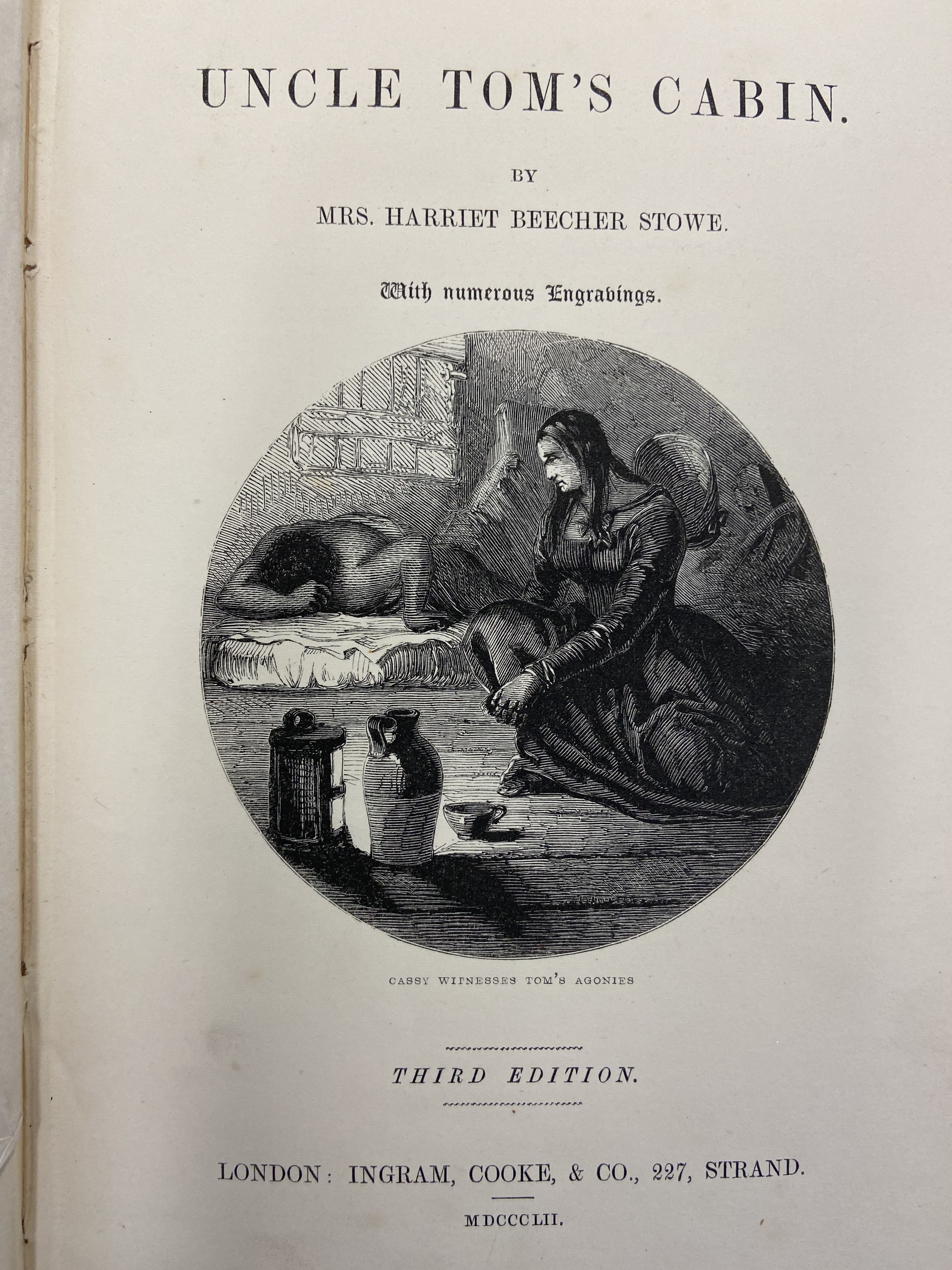This image showcases the inside cover page of the third edition of the book "Uncle Tom's Cabin" by Mrs. Harriet Beecher Stowe, published in 1852 by Ingram Cook & Co, located at 227 Strand, London. The title "UNCLE TOM'S CABIN" is prominently displayed at the top in a serif, all-capitalized font. Below the title, the author's name, "Mrs. Harriet Beecher Stowe," is also printed, and it is noted that the book contains numerous engravings. The center of the page features a circular engraving depicting a woman named Cassie witnessing the agonies of Tom, a black man lying on his stomach on a cot. In the background, various objects such as a jar, a lantern, and a cup can be identified. The woman appears distressed as she looks at the suffering man. Beneath the engraving, the caption reads "Cassie Witnesses Tom's Agonies." Further down the page, in a similar serif font, it mentions "Third Edition." At the very bottom, the publication details, "London, Ingram Cook & Co, 227 Strand" are provided along with the Roman numerals "MDCCCLII," signifying the year 1852. The page appears to be made of paper, suggesting it may be the first page rather than a hard cover.